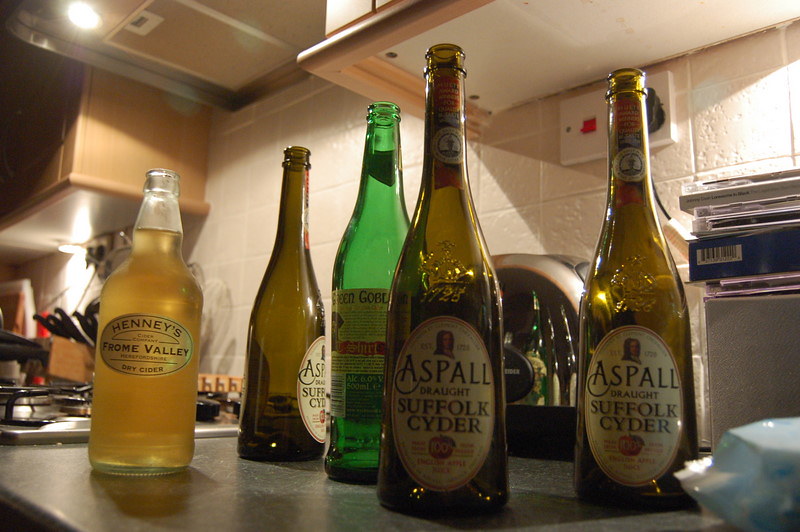The photograph depicts a residential kitchen's countertop adorned with five glass bottles of hard cider. Starting from the left, there's a full bottle of Henny's Frome Valley Dry Cider with a distinctive gold oval label. Adjacent to it stands a green bottle with its label facing away, making the details indiscernible. Centrally positioned and covering a predominant part of the image are two Aspall Suffolk Cider bottles with their labels prominently visible. Further to the right, there's another Aspall bottle, making a total of three Aspall bottles, all of which appear empty. Behind this arrangement, the kitchen background reveals a stove with a visible range, a knife block, and the lower side of the overhead cabinets. Additionally, a toaster can be seen slightly in the background to the right of center. The photographer has positioned themselves such that the bottles' details and labels are in sharp focus against the kitchen setting.